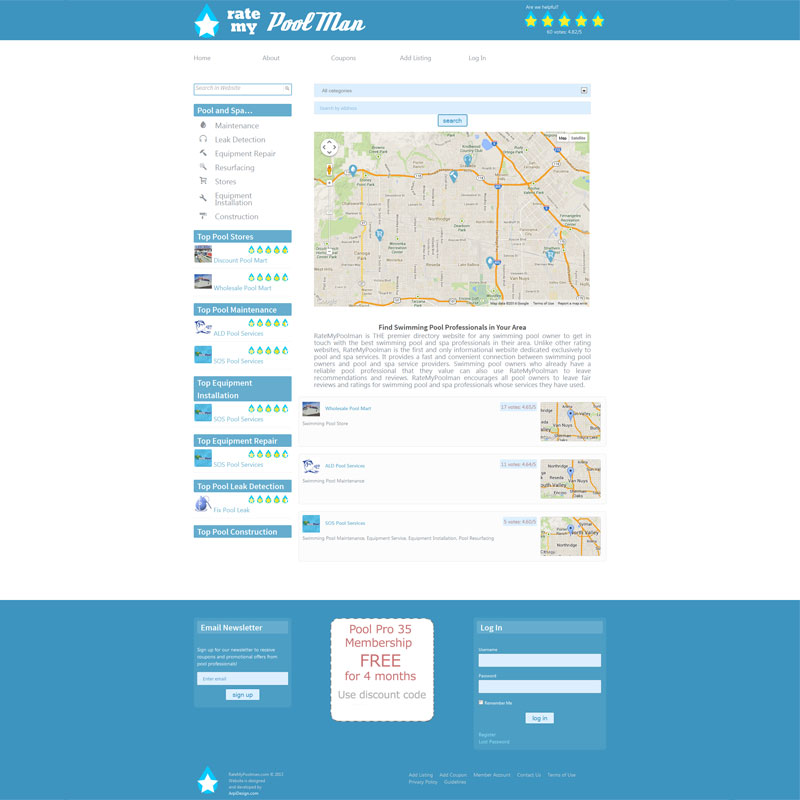This detailed caption provides an overview of the screenshot from the "MyRaidVulman" platform, capturing its various sections and features:

---

"Screenshot from the 'MyRaidVulman' platform displaying various features for finding swimming pool professionals in your area. The main title, 'Find Swimming Pool Professionals in Your Area,' is displayed in black font above a detailed paragraph. Below the paragraph, the interface is divided into three sections displaying different services.

1. The first section features a landmark with a slightly blurry image, accompanied by a rating of 4.68% based on 17 votes. 
2. The second section highlights food services, containing 11 reviews with a rating of 4.64%, alongside a corresponding map.
3. The third section lists 'CQ's Peace Post Services,' showing a rating of 4.60% from 3 votes, also with an accompanying map.

At the bottom of the screenshot, a dark blue footer contains three distinctive boxes:
- The left box, almost translucent, prompts users to sign up for an email newsletter.
- The center box, set against a solid white background, features red text offering a promotion: 'Pool Pro 35 Membership free for four months. Use this code' in gray text.
- The right box, transparent, serves as a login area with fields for username and password, along with a login button."

---

This caption provides a comprehensive description, helping viewers understand the content and layout of the screenshot from "MyRaidVulman."